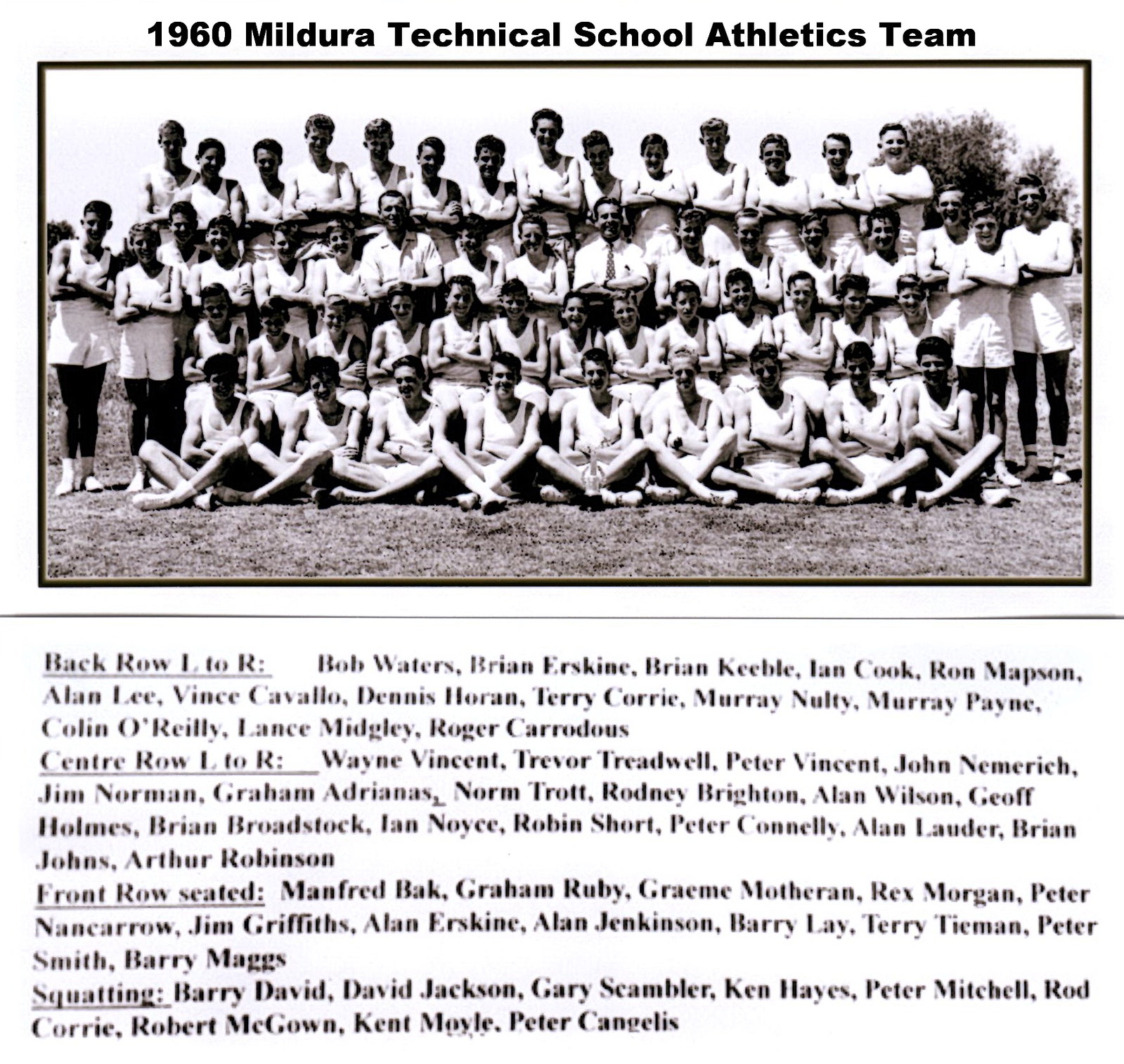The black and white photograph titled "1960 Mildura Technical School Athletics Team" depicts an organized group of approximately 50 men and one woman, positioned in four distinct rows on a grassy field. In the front row, roughly 10 individuals are seated cross-legged, while the second row consists of seated members. Behind them, a third row stands at a lower level, and the back row includes those elevated on some form of stand, enhancing their visibility. The team is uniformly dressed in white outfits, predominantly white shirts or tank tops, and likely white pants. The background features a singular tree to the left and a blank sky, emphasizing the team's setting in an outdoor field. The photograph is framed with a thin black outline and complemented by text above and below. The top text reads "1960 Mildura Technical School Athletics Team," while the bottom text provides a detailed key to the individuals in the photo. This key categorizes the members by their row positions—back row, center row, front row seated, and squatting—each followed by a list of names such as Bob Waters, Brian Erskine, Barry David, and David Jackson. Each category is underlined, maintaining a clear and organized structure on a white background with black text.